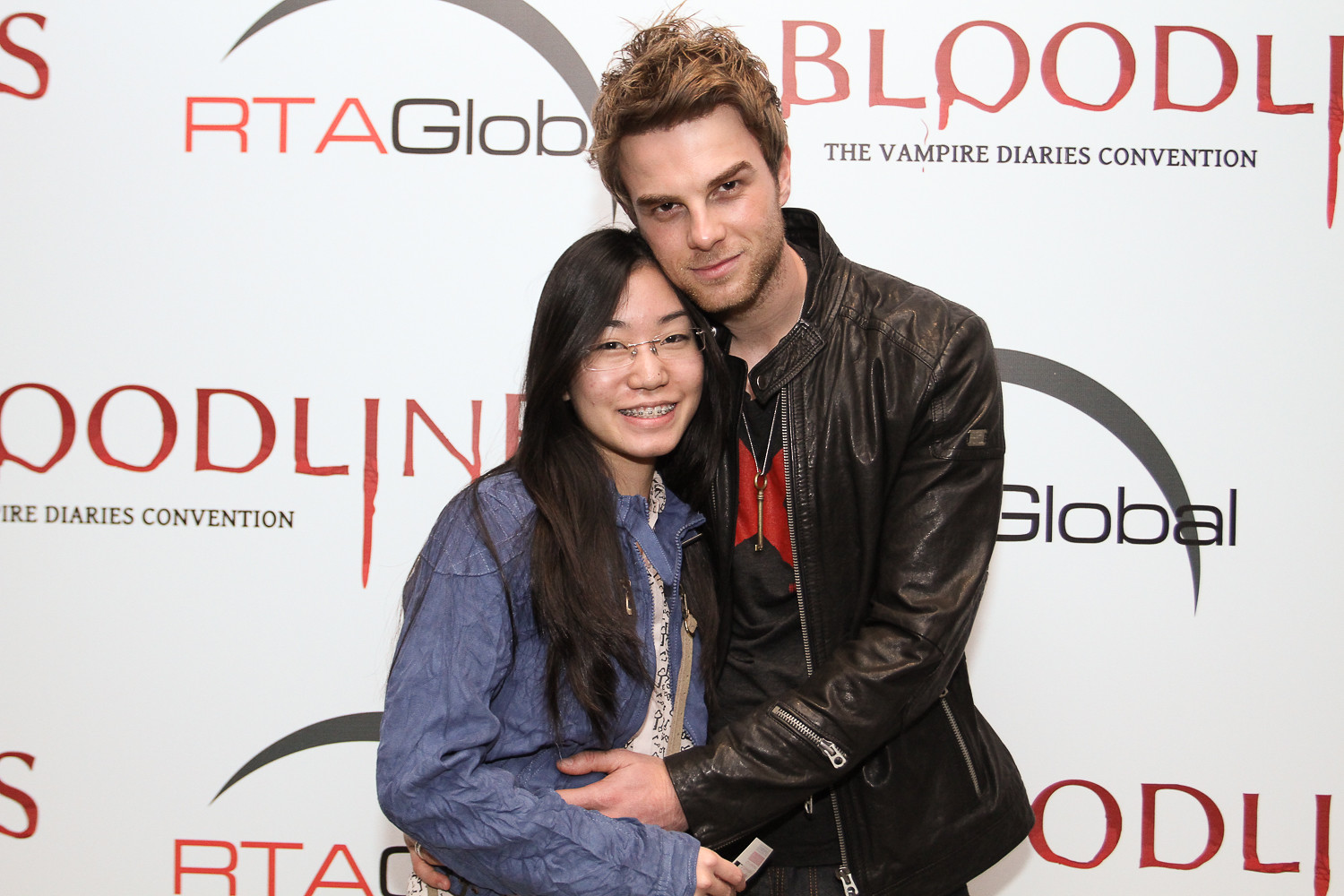In this detailed photograph, two individuals are posing in front of a white backdrop adorned with repeating logos and text including "Bloodlines," "The Vampire Diaries Convention," and "RTA Global," featuring designs of crescent moons. The pair includes a younger Asian woman in her teens, with long black hair cascading past her shoulders. She is wearing rectangular glasses and braces, and she sports a denim jacket over a white blouse with some lettering visible. In her hand, she holds a small gray device, possibly a mobile phone, and she is warmly smiling. Leaning into her, and holding her from behind, is a white man in his late 20s. He has a stubble beard and slicked-back brown hair with subtle blondish highlights. He is clad in a black leather jacket over a black t-shirt that has a hint of red on the chest, and he wears a key necklace around his neck. He gazes at the camera with a smirk, creating a cozy, affectionate scene against the convention-themed backdrop.